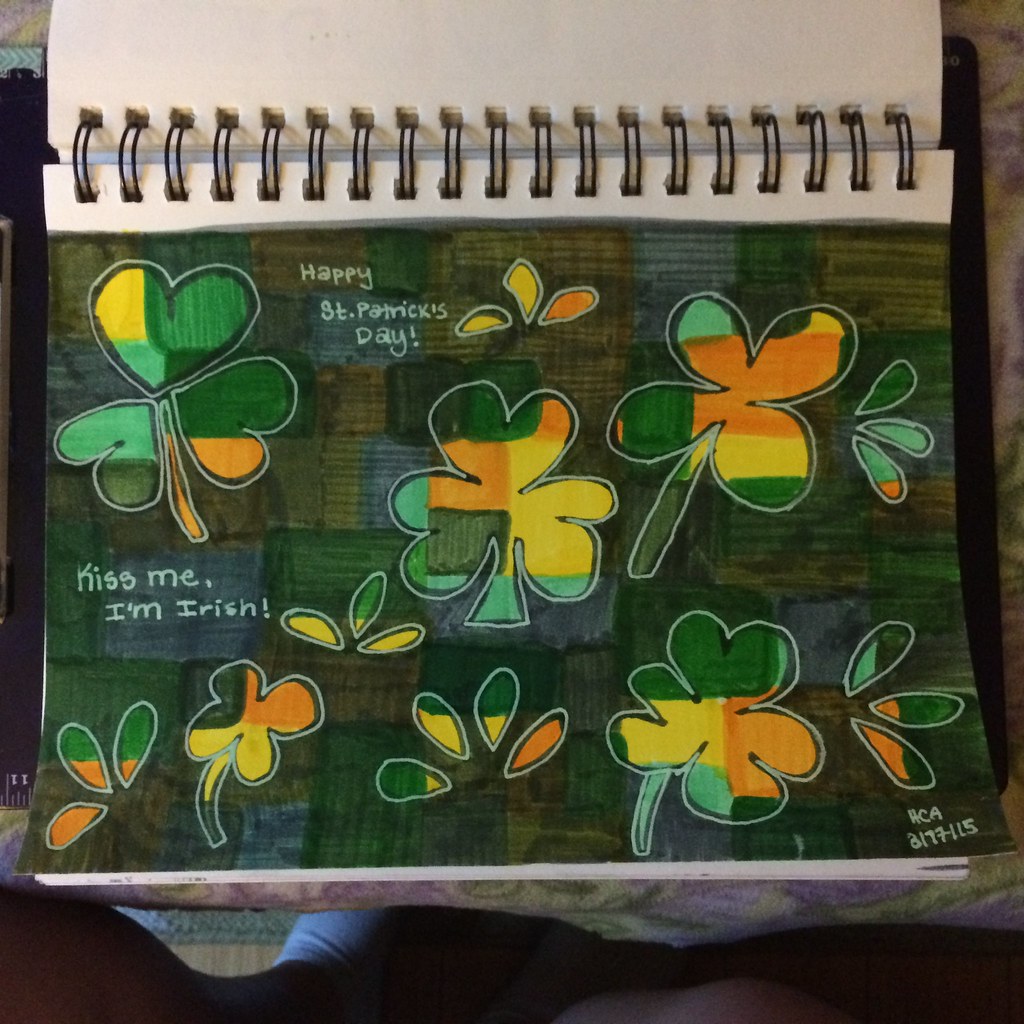This image features a sketch pad that appears to also function as a calendar, mounted on a spiral binding. The sketch pad is adorned with various green clovers, including both three-leaf and four-leaf varieties, along with petals scattered across the page. The background comprises a checkerboard pattern of dark green, olive green, and gray boxes. The prominent text, written in white, reads "Happy St. Patrick's Day" and "Kiss me, I’m Irish." Additionally, there is an alphanumeric code "RCA 3 7 3 line 7 7 - LL 5" inscribed on the page. The sketch pad rests on a pink and purple floral patterned comforter, and a wooden floor and a wall can be seen in the background.